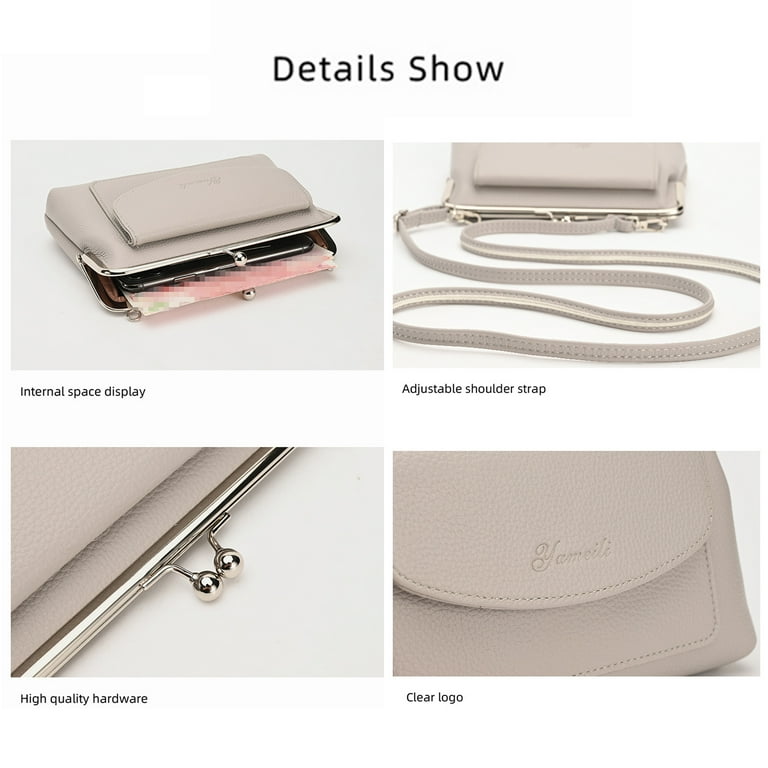This image is a detailed advertisement for a beige, leather-textured purse, split into four photographs to highlight various features. The overall image is labeled "Detail Show" at the top. The top left photo, captioned "Internal Space Display," shows the purse slightly open to reveal an internal compartment, suggesting it can hold items like cards, a phone, and receipts. On the top right, the "Adjustable Shoulder Strap" caption points out the bag’s thin, same-colored, shoulder-length strap, emphasizing its adjustable nature. The bottom left image, captioned "High-Quality Hardware," offers a close-up of the silver metal ball clasp that secures the purse, described as white-gold colored. Finally, the bottom right photo, labeled "Clear Logo," shows the logo "Yameli" engraved into the purse's leather-like material.